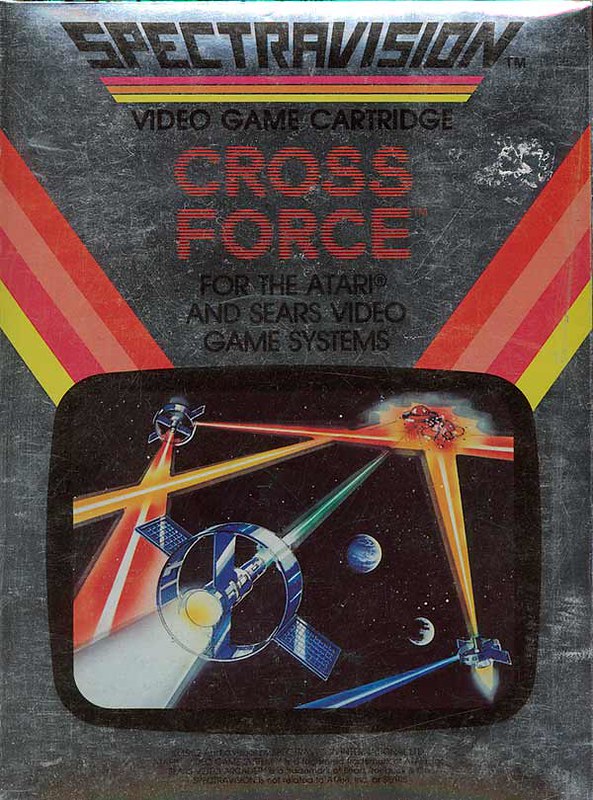This image features a vintage sign for SpectraVision, primarily in black and gray tones with touches of white. The word "SpectraVision" is prominently displayed in bold black letters above three linear accents in red, orange, and yellow. Below, the sign proclaims "Video Game Cartridge" and mentions the title "Cross Force," specifying its compatibility with Atari and Sears video game systems, indicating the image's nostalgic value.

Central to the image is a square depiction of an outer space battle scene. A futuristic spaceship, resembling the rounded part of a propeller, emits a powerful beam of light, symbolizing its destructive force. The vibrant explosion is characterized by beams in vivid red, yellow, green, and blue against a stark black starry background. The cosmic vista portrays two planets, one of which is dramatically splitting into two pieces. Emerging diagonally from this fragmented planet are dynamic stripes in shades of red, lighter red, pink, and yellow, accentuating the explosive action and adding visual momentum to the image.